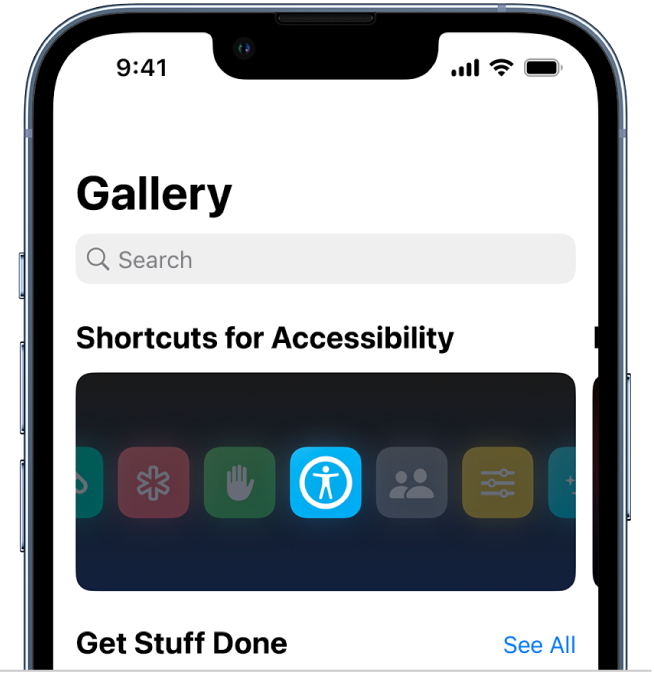The image depicts a cell phone display with a user interface open, showcasing detailed screen elements. The cell phone itself features a black border around the screen, with the time displayed at 09:41 in the top left corner. Adjacent to the time, in the top right corner, are icons indicating signal strength, Wi-Fi connectivity, and a fully charged battery.

The main screen has a white background with "Gallery" as the top heading. Directly below the heading is a grey search bar featuring a magnifying glass icon and the word "Search." Beneath the search bar, the text "Shortcuts for Accessibility" is displayed.

Central to the screen is a rectangular block with a very dark, almost black background, containing seven icons arranged in a straight line across its middle. There are five fully visible icons and two partially visible ones. The center icon, highlighted in light blue, features a white circle with a white stick figure inside it. Below this highlighted icon, the text "Get Stuff Done" is displayed. To the right, the words "See All" appear as a clickable option.